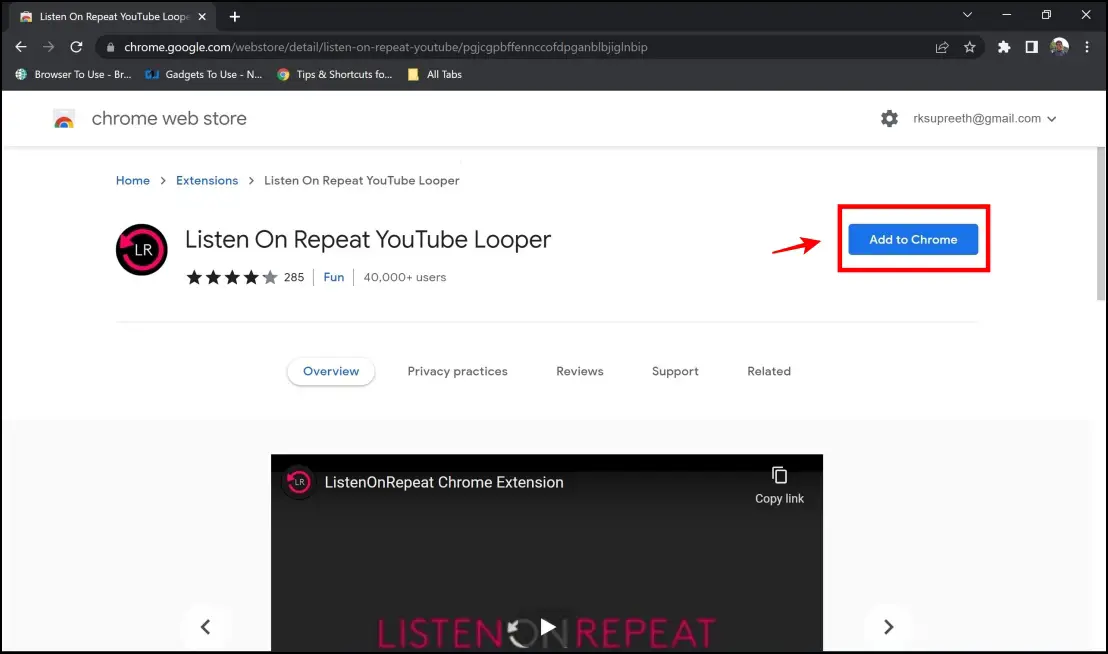This image depicts a detailed screenshot of the Chrome Web Store page for the "Listen on Repeat YouTube Looper" extension. At the top is an active gray-highlighted browser tab. Below this is a horizontal black bar containing several white icons: a plus symbol on the left, followed by a drop-down arrow, a minus symbol, a box, and an "X" on the right. 

Below the black bar is a gray address bar featuring navigation buttons including a white left-pointing arrow, a white right-pointing arrow, a refresh icon, and a black address bar. The address bar displays the URL "google.chrome.com/webstore/detail/listen-on-repeat-YouTube". Adjacent to the URL field is a star icon for bookmarking, a puzzle piece icon, another white box, and a user icon with a profile picture.

The header section beneath the address bar displays a greenish circle on the left side with the words "browser to use" in white, followed by a blue box labeled "gadgets to use N". Next to these, the Google logo is visible, characterized by its green, red, yellow, and blue colors, and the text "tips and shorthand" in white. Adjacent is a yellow box labeled "all tabs". Below this header, the text "Chrome Web Store" appears in black, with a gear icon to its right. 

Further down, a navigation menu is shown with "home", "extensions" in blue, and "listen on repeat YouTube looper" in black. An icon comprising a black circle with the letters "LR" in white and a red semi-circle is beside the title “listen on repeat YouTube looper”. To the right of this, a prominent blue button labeled "Add to Chrome" is encircled in red, with a red arrow pointing to it.

The section under this shows tabs for "overview" in blue, "privacy practices", "reviews", "support", and "related" all in black, leading into a black content area. Centered at the top of this black content area, white text reads "listen on repeat Chrome extensions", with the main title "listen on repeat" displayed in pink and white lettering below, emphasizing the "on repeat" part in red.